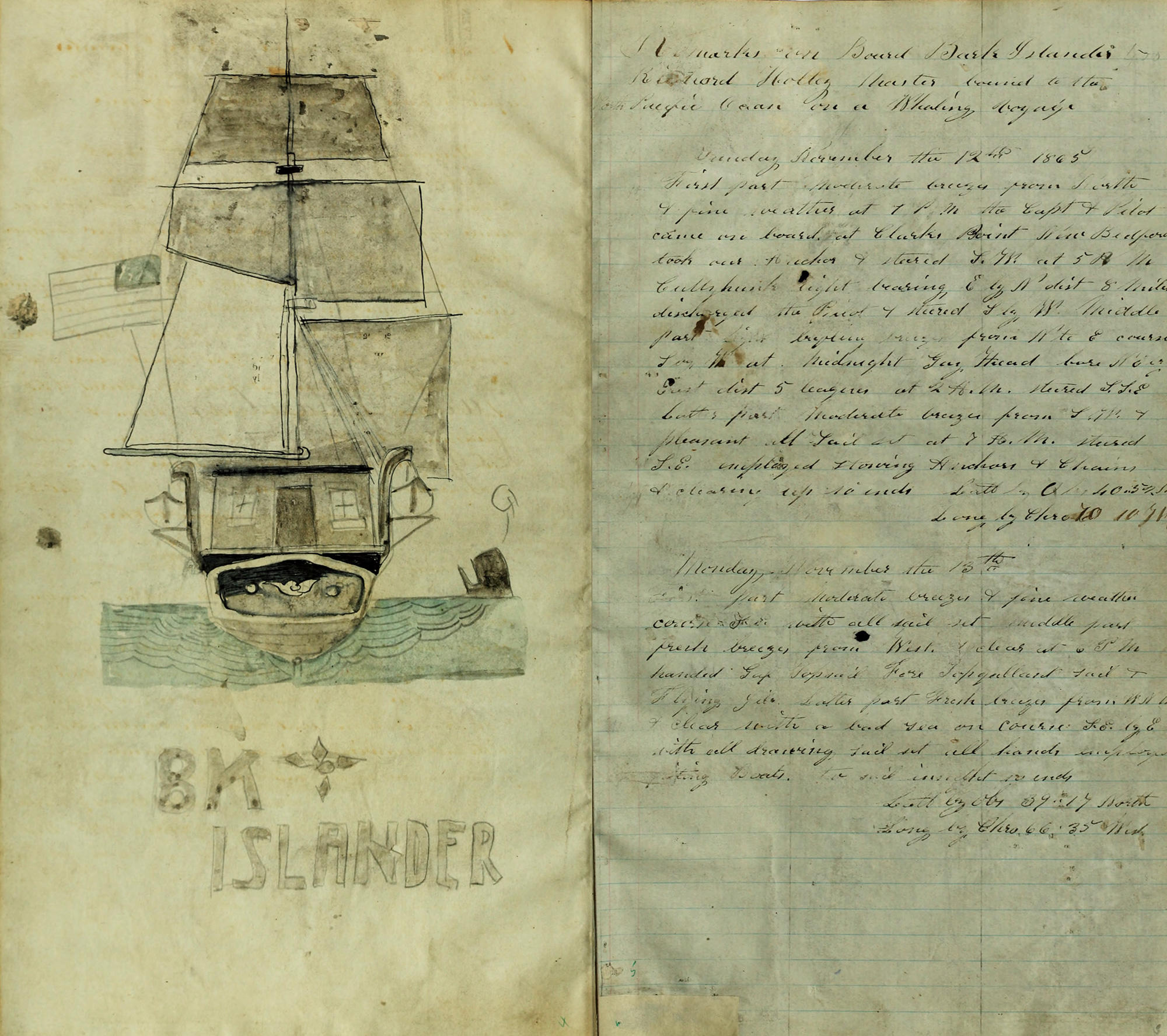The image displays two aged and crumpled pages, reminiscent of an old journal. The left page features a hand-drawn, colored illustration of a large sailing ship from the Age of Sail, with several extended sails. An American flag flutters from the left side of the vessel. Sailing towards the viewer, the ship is labeled "B.K. Islander" in handwritten text below it. The blue sea beneath is decorated with a simplistic, almost cartoon-like whale rising from the water. The right page comprises about 30 lines of intricate and precise cursive script, written on lined paper. Although the writing is difficult to decipher, it is beautifully executed, suggesting a meticulous hand. Both pages reveal significant age-related wear, indicating their historic nature.